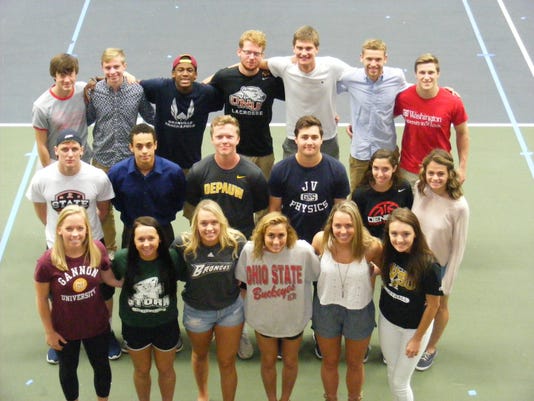Aerial photograph of a large group of predominantly college-aged students standing on an outdoor tennis court with a green and gray surface marked by white lines. The back row consists of seven men, the middle row features four men followed by two women on the right, and the front row includes six women, two of whom, positioned on the ends, are wearing long pants while the others are in shorts and t-shirts. Notable shirt logos include universities such as Gannon University, Ohio State, DePauw, and Washington University. The photograph shows an array of colors, including red, dark blue, black, orange, maroon, white, and yellow, predominantly on their shirts. The overall focus is on the group centered within the court, highlighting the diverse academic affiliations and casual, sporty attire.